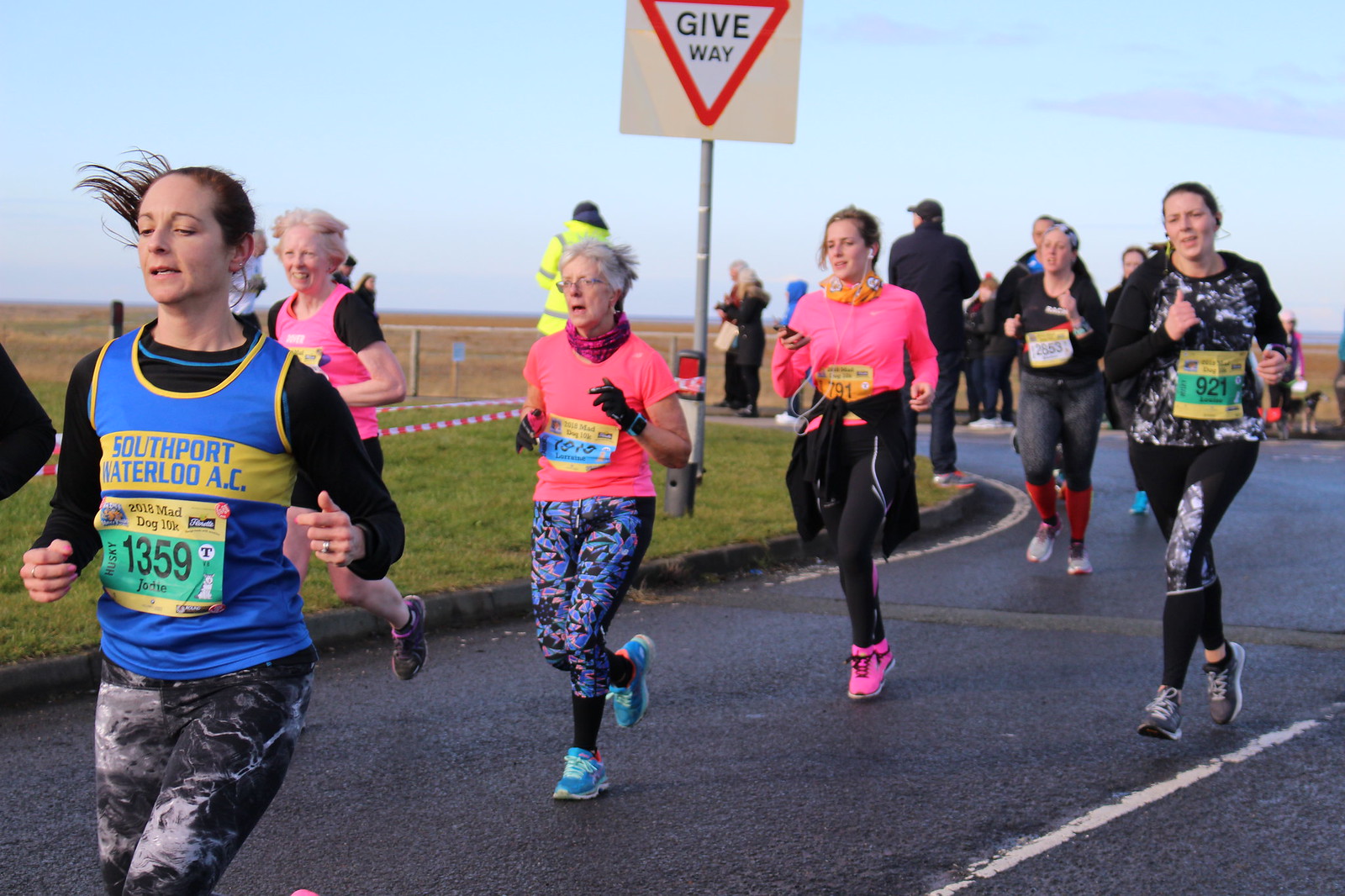This photograph captures an all-female racing event, likely a marathon or charity run, held on a damp asphalt road bordered by green grass. The image shows approximately 10 to 15 participants, with a clearer focus on about 12 runners. Most runners don long-sleeved jogging suits and running shoes, indicating cooler weather. At the forefront, a middle-aged woman wearing a blue jersey with the text "Southport Waterloo AC" and the number 1359 leads the pack. Flanking her are two older women in pink tops, followed by younger runners. The black road, marked with a white line, snakes through flat plains under a clear blue sky, making it a scenic daytime event. A security guard looks on from the sidelines, and in the background, a "Give Way" street sign with a distinctive red-outlined, upside-down triangle stands amidst the grassy verge. The ground appears wet, suggesting recent rain, adding an extra challenge to the race.